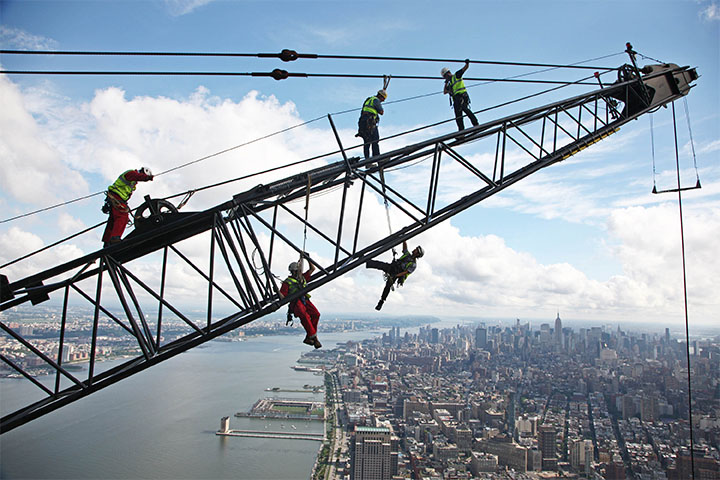The image captures a dramatic scene of five construction workers executing their tasks atop a towering crane, suspended high above a sprawling urban landscape. The workers, all equipped with hard hats and neon safety vests, are divided between two distinct positions: three are perched atop the crane, while two are visibly hanging from below, secured by safety harnesses. The crane itself slices diagonally through the image, extending from the bottom left to the top right. The backdrop features a bustling metropolis characterized by an array of skyscrapers that dominate the foreground, juxtaposed by the serpentine flow of a wide river or possibly an ocean inlet. The high vantage point of the photograph offers a panoramic view, revealing the tops of numerous buildings and extending to a tranquil sky dappled with fluffy white clouds, suggesting a clear and sunny day.